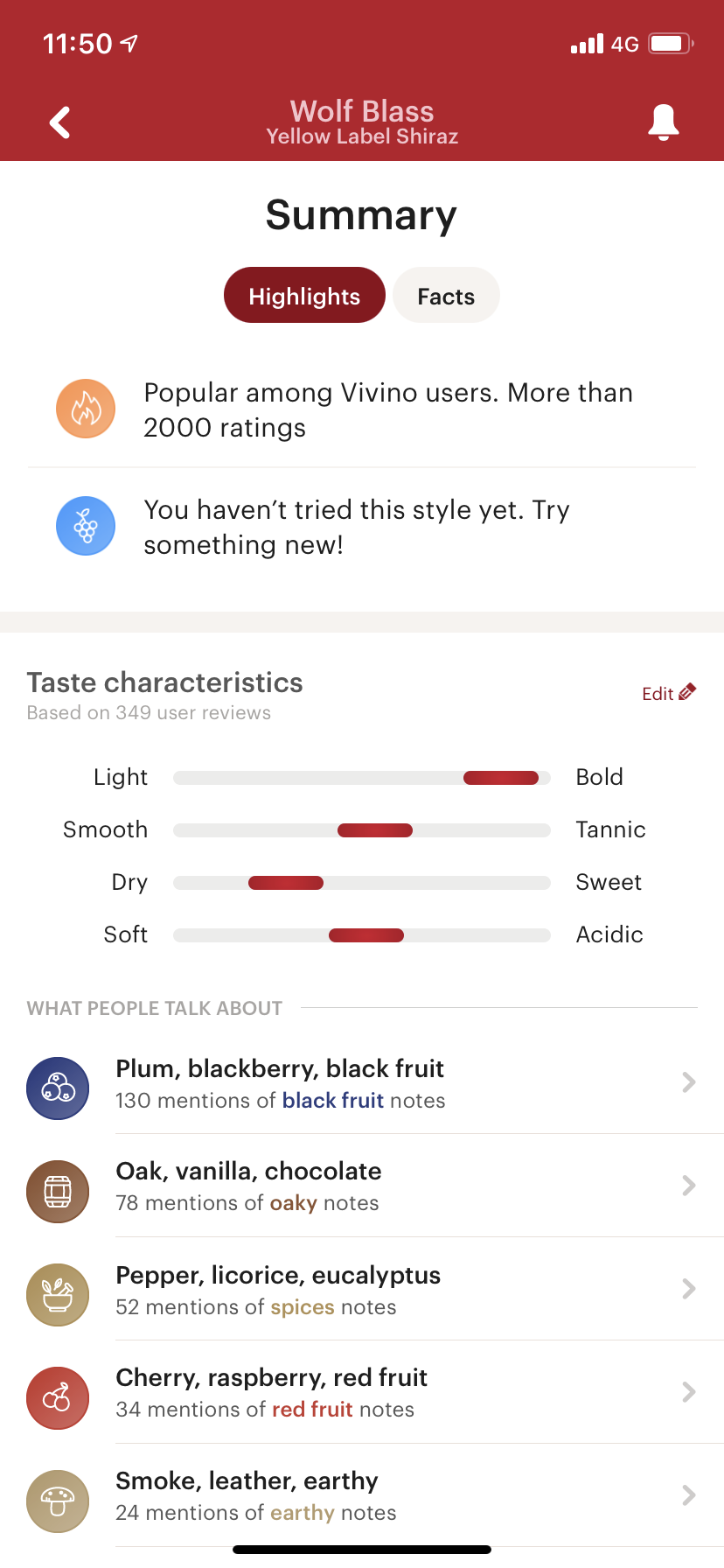This image is a detailed screenshot from a mobile application, showcasing a variety of wine-related information. The topmost section features a red header with a centered gray text displaying "Wolf Blass Yellow Label Shiraz." Adjacent to this text, there's a white arrow pointing left on the left-hand side and a white bell icon on the right-hand side.

Below this header, the interface features a white background with "Summary" written in bold black text. Directly beneath, users can see two prominent, rounded buttons: one on the left in red with white text stating "Highlights," and one on the right in light gray with gray text labeled "Facts."

The content area is divided into distinct sections, demarcated by thin gray lines. The first section titled "Popular Among Vivino Users" highlights that the wine has gathered more than 2,000 ratings. This section is ornamented on the left by an orange circle featuring a white fire icon. 

The subsequent section encourages exploration with the text "You Haven’t Tried This Style Yet. Try Something New," paired with a blue circle containing a white grape icon.

A thick light gray line distinctly separates this part from the next section, which is labeled “Taste Characteristics” at the upper left corner against a white background. Subtext in small light gray reads, "Based on 349 User Reviews." Adjacent to this, a small red text saying "Edit" accompanied by a red pencil icon is positioned to the right.

The taste characteristics are conveyed through four horizontal scales, each represented by a light gray line with a red, pill-shaped indicator highlighting the position on the scale. The first scale is labeled "Light" on the left and "Bold" on the right, with the indicator near the "Bold" end. The second scale ranges from "Smooth" to "Tannic," with the marker slightly right of center. The third scale contrasts "Dry" on the left and "Sweet" on the right, with the pill around three-quarters towards the "Dry" end. The final scale spans from "Soft" to "Acidic," with the indicator centered.